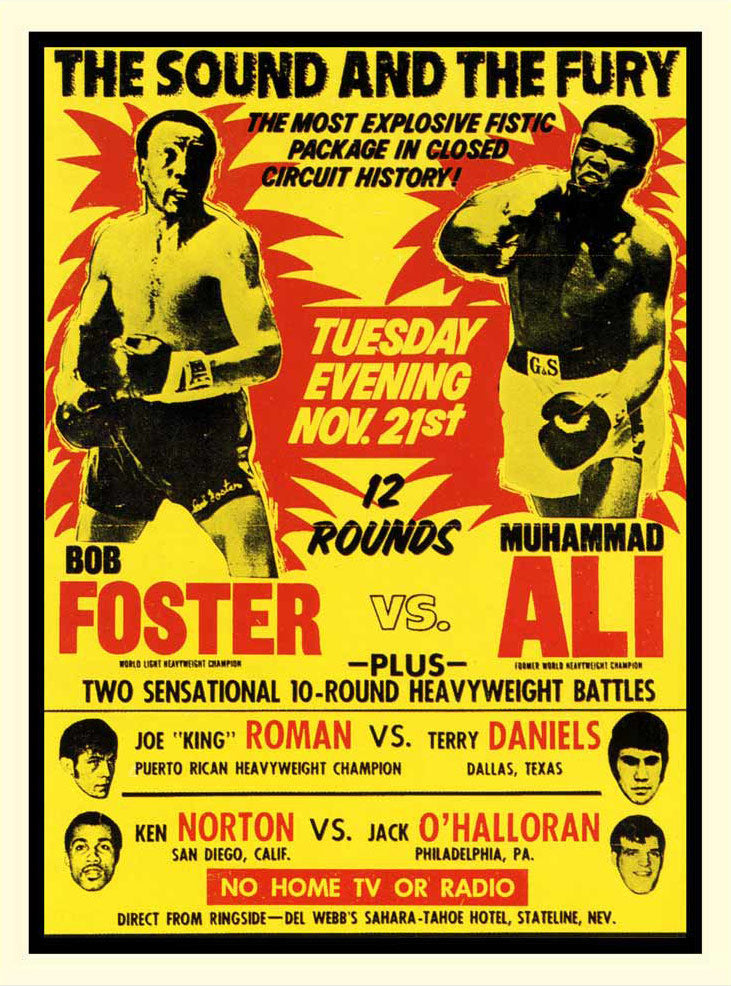The image is a vividly detailed poster for a historic boxing event. Dominated by a striking yellow background with red accents, the poster features prominent images of the two main fighters in action: Bob Foster on the left and Muhammad Ali on the right. The top of the poster boasts the tagline "The Sound and The Fury: The Most Explosive Fistic Package in Closed Circuit History." Between the fighters' names and images, the poster details the main event: "Tuesday Evening, November 21st, 12 Rounds." 

Below this, the poster highlights two additional 10-round heavyweight battles: Joe King Roman, touted as the Puerto Rican Heavyweight Champion, versus Terry Daniels from Dallas, Texas, with their respective images; and Ken Norton from San Diego, California, versus Jack O'Halloran from Philadelphia, Pennsylvania, also accompanied by their images. The bottom of the poster strictly states, "No Home TV or Radio - Direct from Ringside Del Webb's Sahara Tahoe Hotel, State Line, Nevada," emphasizing the exclusive nature of the live broadcast event.